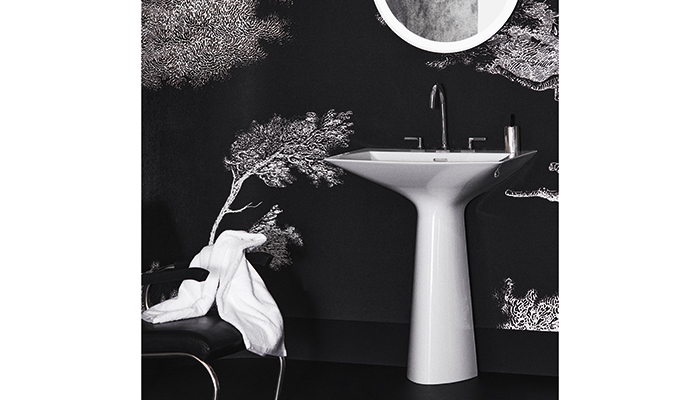This black-and-white photograph depicts an elegantly designed bathroom with a distinct contrast between black and white elements. The background features a black wall adorned with intricate white illustrations of trees, which may either be wallpaper or a potted plant's branches extending into view. Central to the image is a pristine white pedestal sink, slightly off-center to the right, with chrome dual faucets and a sleek silver pump-style dispenser with a black top situated on its right side. Mounted above the sink is a half-visible circular mirror with a white border, cut off by the edge of the square frame. To the left of the sink, a black cushioned chair with two armrests supports a casually draped white towel. The overall sophisticated atmosphere suggests the bathroom could belong to an upscale restaurant.